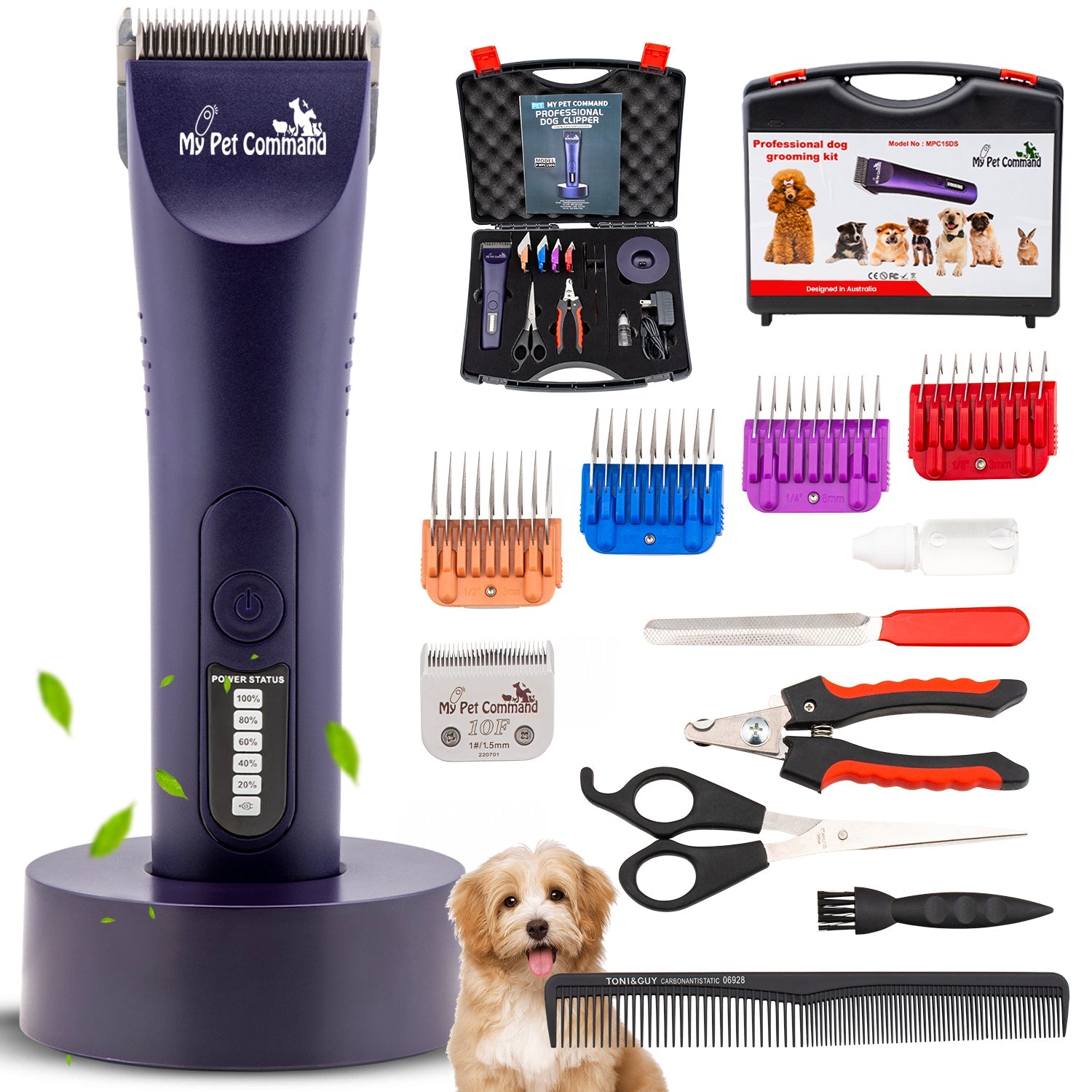The photograph showcases a comprehensive pet grooming kit. Dominating the left side is an electric dog trimmer, standing vertically on a grayish-black base. The trimmer is a purplish color, with "My Pet Command" inscribed below the blades. Adjacent to the trimmer, a smaller image displays the opened black case, revealing the trimmer and its various attachments. To the far right, another smaller picture illustrates the closed case, bearing images of dogs and labeled "Professional Dog Grooming Kit." Below these, four detachable blade tips in yellow, blue, purple, and red are neatly arranged. Beneath the red blade, a small plastic bottle is visible, next to a red-handled nail file, black-handled pliers, black-handled scissors, a small black brush, and a black comb. At the bottom center of the image is a charming photograph of a tan dog with its tongue playfully sticking out.